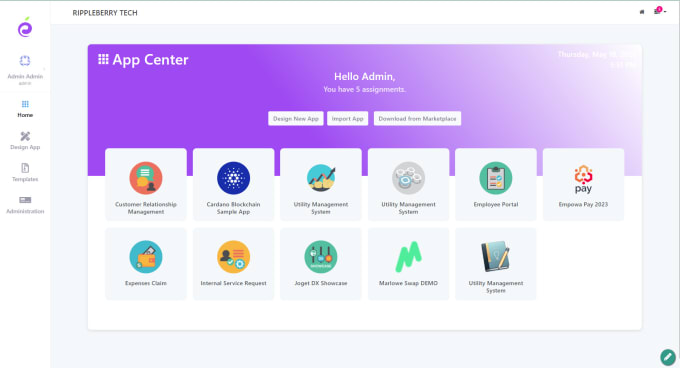The image depicts an application interface on what seems to be a tablet, displayed in a horizontal orientation. It could potentially be a website, though it lacks an address bar, indicating it is likely an app.

In the top-left corner, there is a purple icon with a green element protruding from the top, labeled "admin." Below this icon, the menu options include "Home," "Design App," "Templates," and "Administration," indicating a structured navigation system. Adjacent to this menu, the text "Rippleberry Tech" is displayed, suggesting the name of the application or the organization associated with it.

In the upper-right corner, there is an unidentifiable icon marked with a red circle, possibly indicating a notification or alert.

The main part of the interface is divided into two sections: a purple header and a white body. In the top-left of the purple header, there is a grid icon labeled "App Center." Below it, the text greets the user with "Hello, admin." It also mentions, "You have five assignments," followed by options such as "Design New App," "Import App," and "Download from Marketplace."

Beneath these options, there are various icons representing different tools or modules available in the application. These include:

- Customer Relationship Management (CRM)
- Cardano Blockchain Sampler App
- Utility Management System (appearing three times)
- Employee Portal
- EmpowerPay 2023
- Expenses
- Clare
- Internal Service Request
- JogetDX Showcase
- Marlowe Swap Demo

These modules appear to provide a range of functionalities for managing different aspects of the business or application environment.